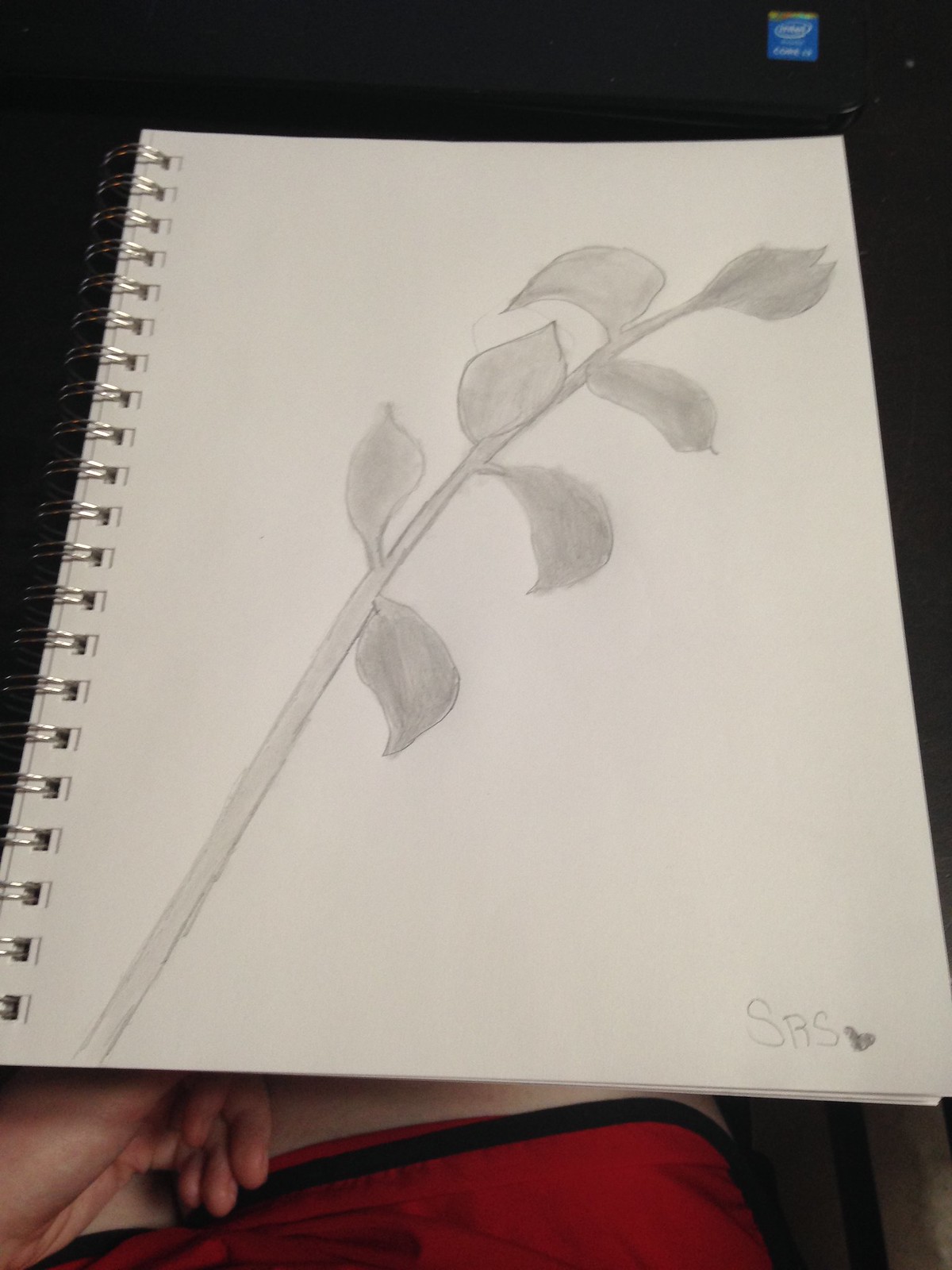The photograph depicts a sketchbook resting on someone's lap, capturing an intimate moment of creativity. Visible in the image are the artist's hand and leg, suggesting a relaxed and casual setting. The sketchbook features an unlined sheet of white paper, bound by spirals on one side. At the bottom of the page, the artist has signed their work with "SRS" and a small heart, adding a personal touch.

The drawing itself is rendered in gray pencil and showcases a beautifully detailed flower with delicate leaves. The flower at the top is shaded in dark gray, contrasting with the lighter gray tones of the leaves. The slender stem is also meticulously colored, reflecting the artist's careful attention to detail. The image is of high quality, capturing every nuance of the sketch.

The person appears to be wearing red shorts with a black trim, further emphasizing the casual and personal nature of the scene.